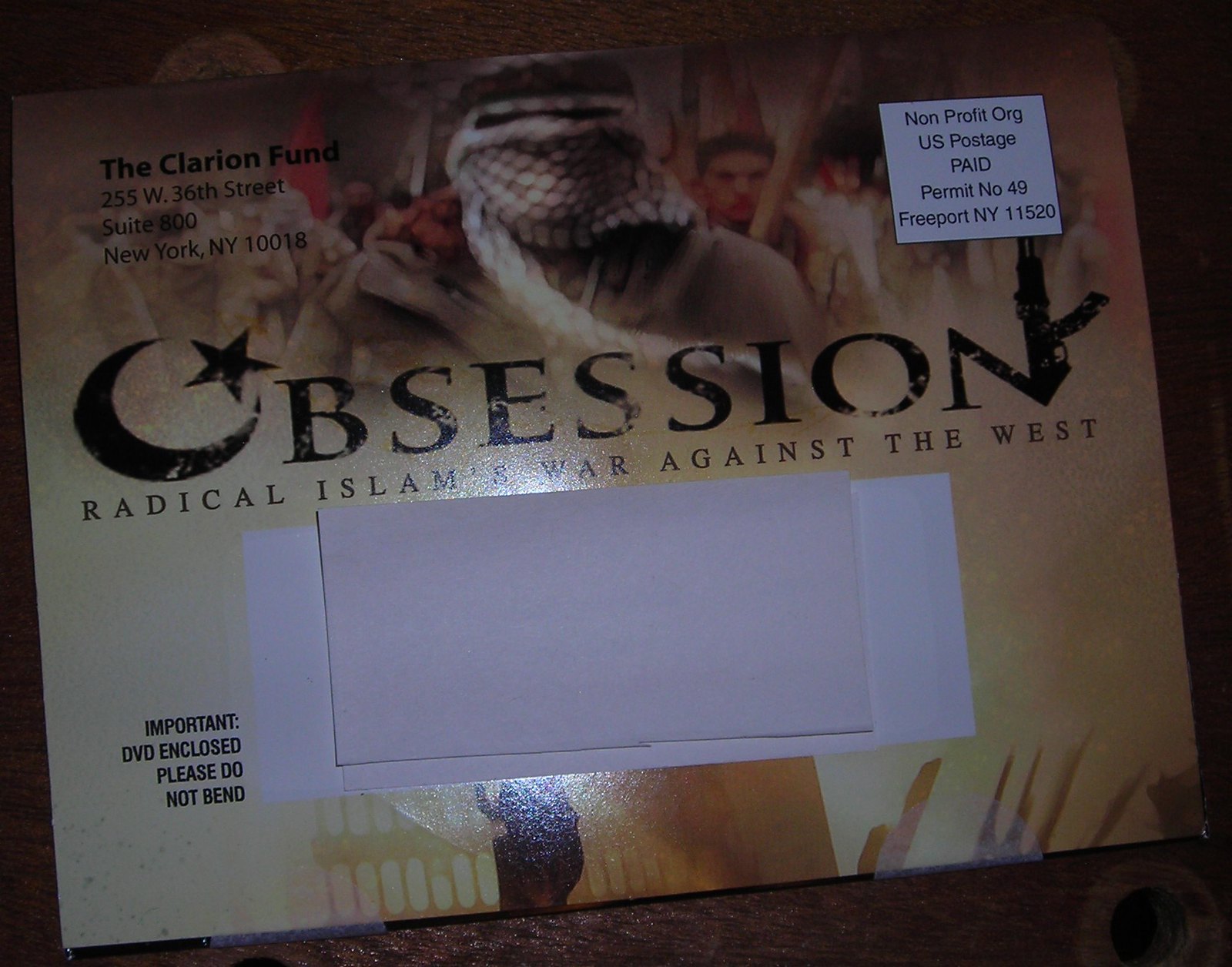This image depicts a glossy, large postcard-style political mailing typically found in mailboxes, primarily from a conservative fundraiser. Dominated by the bold word "Obsession" in the middle, the letter 'O' features the crescent moon and star symbol associated with Islam, while the 'N' is embellished with an illustration of an AK-47 rifle. The tagline "Radical Islam's War Against the West" follows underneath. The background displays a group of individuals, with one prominently shown with his face covered, conveying the image of a terrorist, and other angry men behind him, creating an atmosphere of fear. The top left corner reads "The Declarian Fund, 255 West 36th Street, Suite 800, New York, NY 10018." The bottom left corner prominently states "IMPORTANT DVD ENCLOSED, PLEASE DO NOT BEND" in capital black letters. Additionally, the recipient’s address in the center is obscured by a slip of paper. The overall intent appears to be to provoke a strong emotional reaction, potentially to galvanize fundraising efforts.